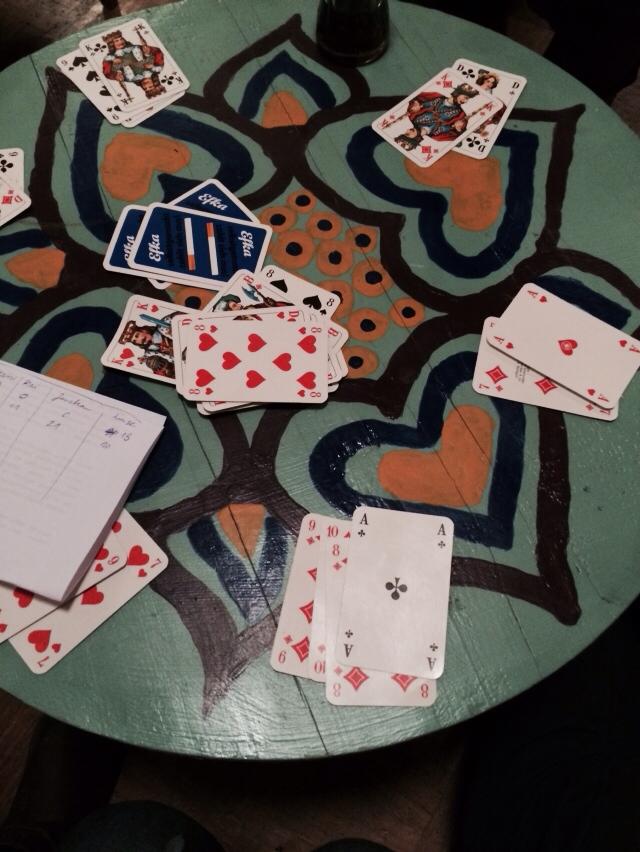In this photograph, a lively card game is taking place over a distinctively painted wooden circular table. The table features a soothing light mint green background with a central design of peach circles adorned by dark purple or brown dots. Encircling these central peach circles are multiple large hearts, each characterized by a brown outer layer, a mid-sized blue heart within, and a smaller peach heart at the core.

The card game in progress is visualized with several scattered piles of cards. At the very center, a stack of face-down cards is noticeable by its blue, white, and orange striped backs, adorned with white lettering. Next to this central pile lies a smaller stack of cards face up. Surrounding these central decks are various smaller piles: closest to the camera is a group of three or four cards, then moving counterclockwise, a pile of two cards is positioned. Continuing clockwise from the initial set, another duo of cards and yet another pair mark the bottom left corner of the table.

Additionally, a pad of white paper lays on the table, featuring hand-drawn columns and numbers, which likely keep track of the game's scores or some other crucial element of gameplay. The overall scene is rich in intricate details, enhancing the sense of engagement and activity inherent in the card game.